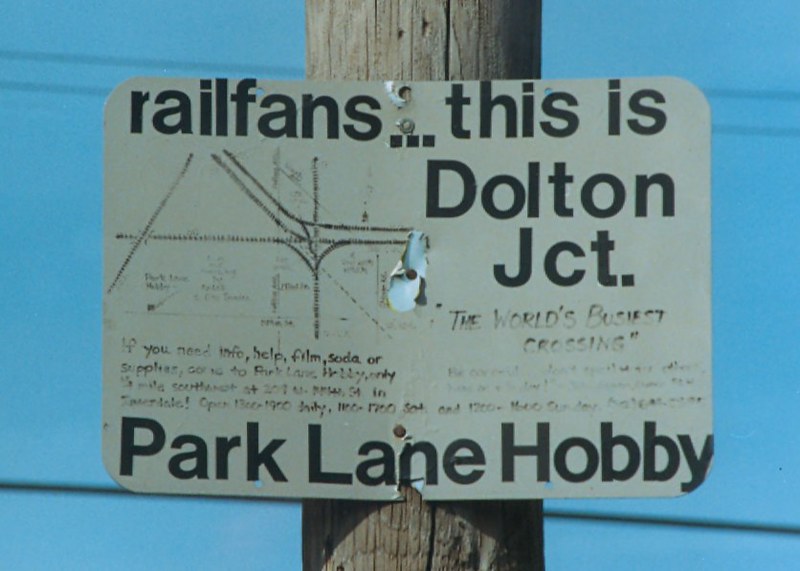In the center of a horizontally aligned rectangular photograph, there's a weathered wooden telephone pole with visible vertical cracks. Attached to the pole is a white metal sign with black print. The top of the sign reads, "Railfans... This is Doulton Junction, the world's busiest crossing." Beneath this text, there is a small, faded diagram, possibly a railway map, and some additional text, worn and difficult to read, detailing help, info, film, soda, or supplies available at a place called Furl. Lower on the sign, it states, "Park Lane Hobby" in large, bold black text. In the background, three blurry telephone cords stretch across a clear, blue sky, two near the top and one near the bottom of the image.